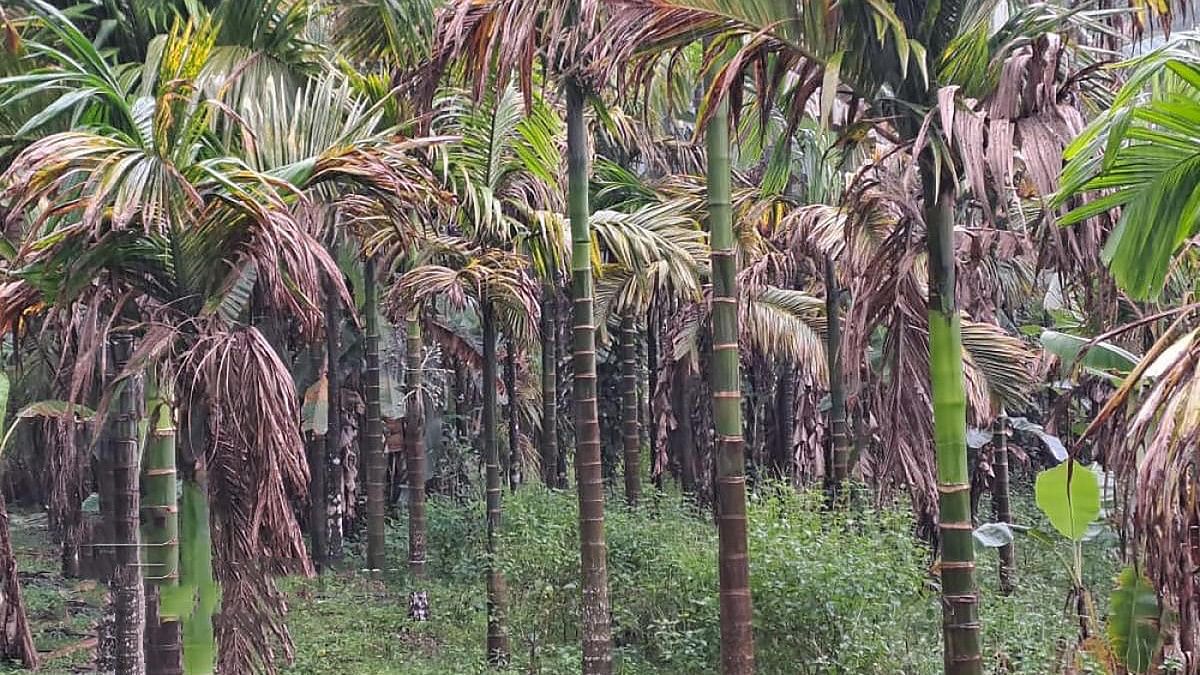The photograph captures a densely packed grove of palm trees in a tropical setting, bathed in natural light and horizontally aligned. The slender, segmented trunks of the trees are predominantly green but show streaks of brown and dry lines, likely from past fronds. A striking feature is a lighter green section on the middle right palm, about three-quarters of the way up, adding a variation in the color palette. The scene is brought to life with green fronds draping in the foreground on the right side, interspersed with hints of yellow and brown, indicating some dried, dying leaves hanging low, while the vibrant, living leaves crown the tops of the palms. Below, the forest floor is carpeted with a mix of green vegetation and foot-high weeds, along with some larger plants boasting thick, green leaves. A diagonal path snakes up from the lower left, where the ground rises slightly higher than the right. This rich and textured image extends vertically, with the foreground showcasing discernible individual trunks, which meld into a dense mosaic of foliage and intertwined tree trunks in the background. The overall ambiance suggests it is a scene captured after the advent of color photography, likely from a lush tropical rainforest.